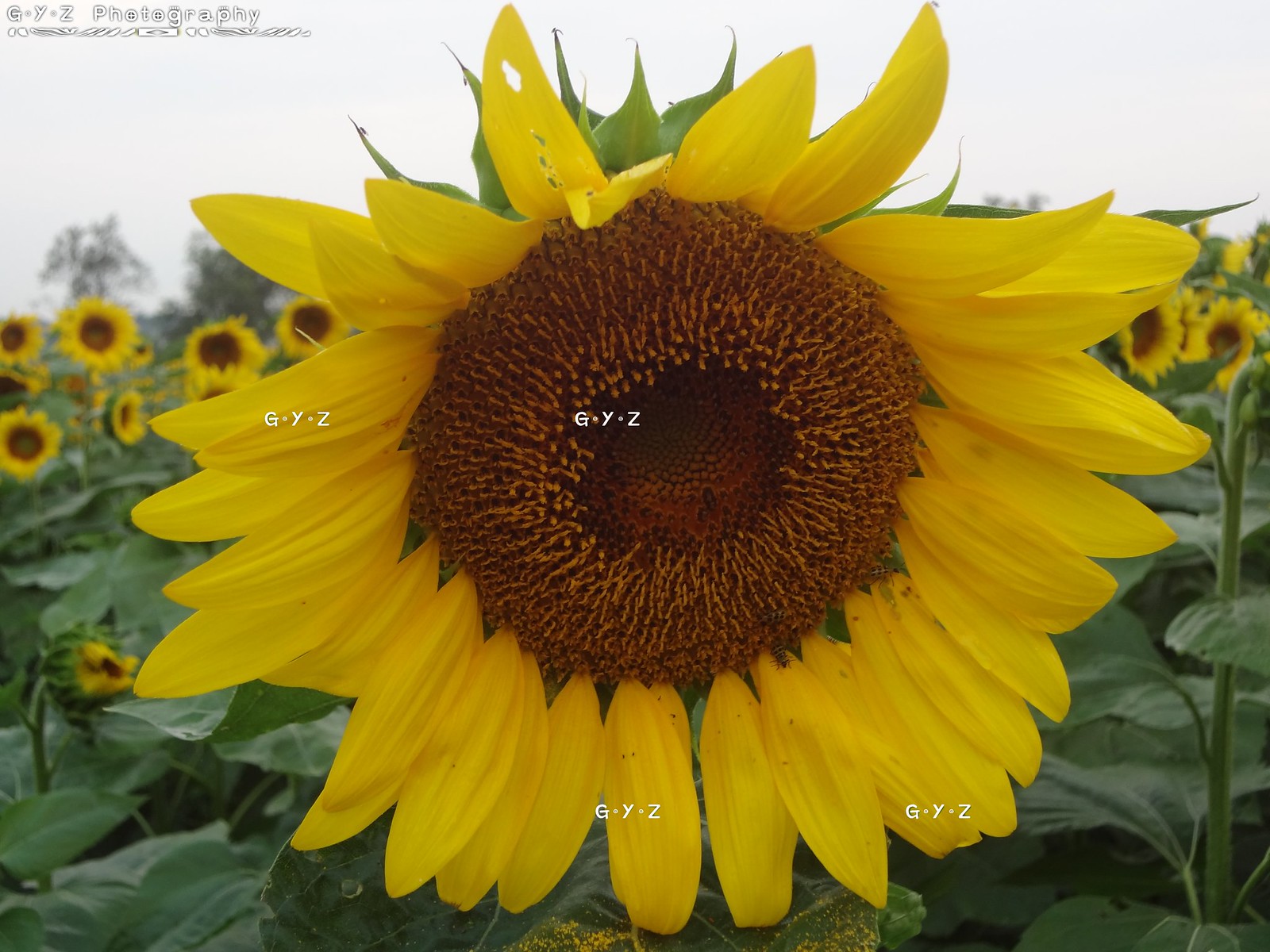In the foreground of this vibrant photograph by GYZ Photography, a colossal sunflower dominates the image with its bright yellow petals and brown, seed-filled center. The petals, delicate and gauzy, encircle the dark middle, with one notable petal at the 11 o'clock position displaying several distinctive holes, revealing the green foliage beneath. The perspective, likely captured with a curved lens for an exaggerated effect, places this singular sunflower front and center, making it appear gigantic against a backdrop of identical sunflowers that gradually fade into the background. Below, the lush green leaves of the sunflowers blanket the scene, while above, a strip of white sky and a faint tree on the far left complete the setting. Numerous faint GYZ watermarks are scattered throughout the image, including one on the center of the sunflower, subtly blending into the vibrant details of the flower. The photograph exudes a rich, textured beauty, capturing the essence of a field immersed in golden blooms under a bright, serene sky.